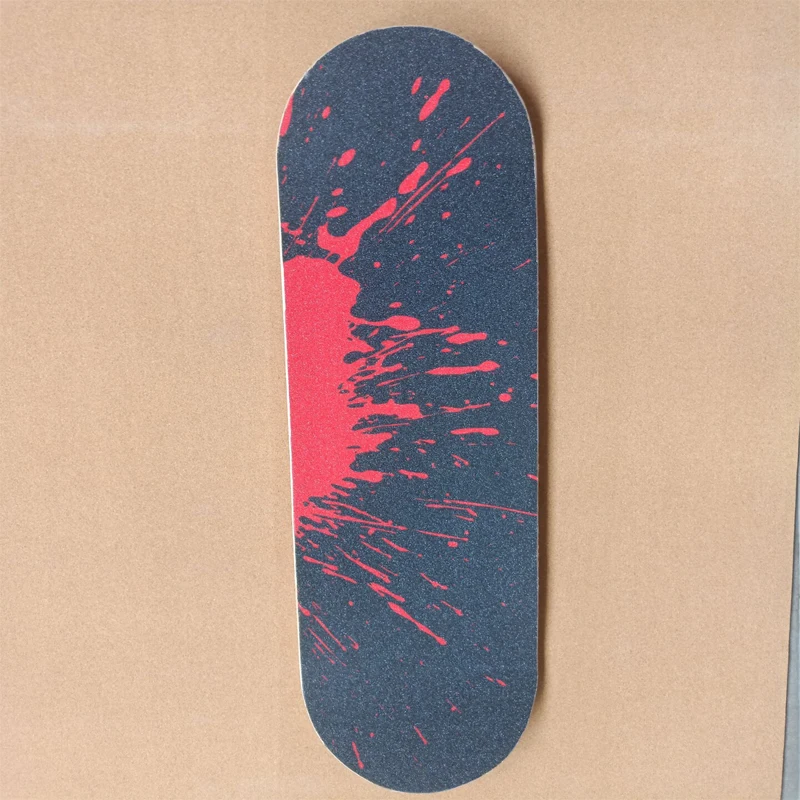This is a detailed color photograph of a skateboard positioned vertically on a surface that resembles light tan butcher paper. The skateboard, viewed from above, displays its grip tape, which is a rough, sandpaper-like surface in charcoal gray. Dominantly, there's a vibrant splash of red paint located on the left side, stretching across the middle half and scattering smaller droplets towards the right side. The bold red contrasts strikingly with the dark grip tape, and the rough texture mimics that of the background surface, creating a coarse aesthetic. The photograph captures the skateboard's shadow on the right, hinting at the lighting direction and adding depth to the image. The skateboard spans from the bottom to the top of the picture, emphasizing its central placement and vertical orientation.